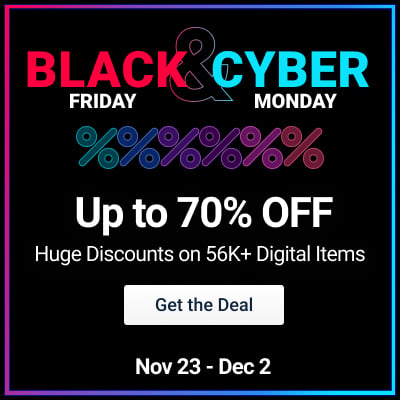This advertisement features a striking black background with a vivid, gradient frame that transitions from fuchsia to purple to teal, then a deeper teal, back to purple, and finally returning to pink. At the top, bold text reads "Black & Cyber." The word "Black" is rendered in red, while the larger ampersand is only outlined, and "Cyber" appears in teal. Beneath "Black" and "Cyber," the words "FRIDAY" and "MONDAY" are displayed in white, all capital letters, respectively. 

Below these labels are six colorful percentage signs in shades of green, blue, purple, red/purple, pink, and red. Following this, a prominent message in white, all capital letters declares, "UP TO 70% OFF." Accompanying this are smaller letters specifying huge discounts on over 56,000 digital items. A white box with black text urges viewers to "GET THE DEAL," and the promotional period is noted as spanning from November 23rd to December 2nd.